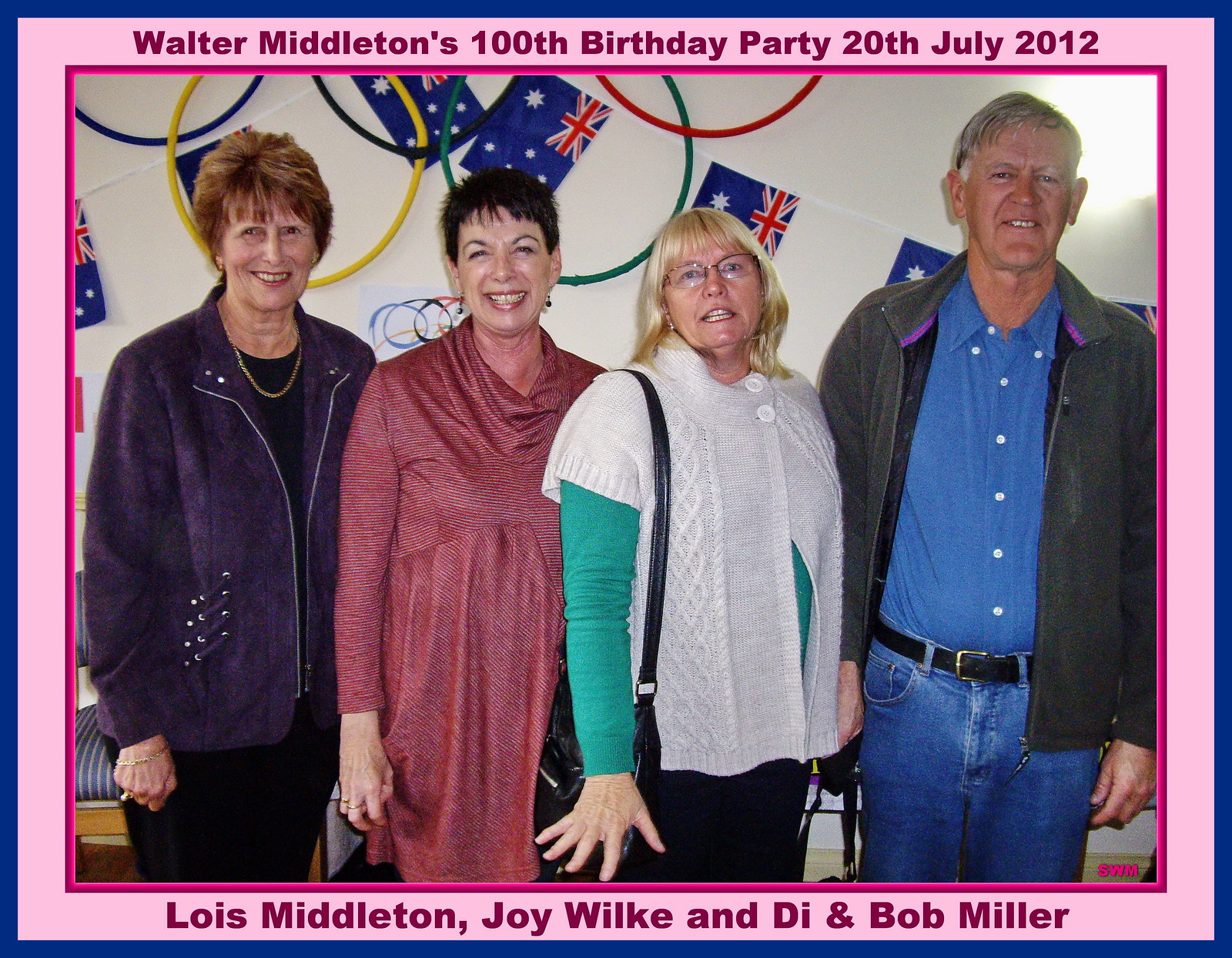This is a color photograph taken at Walter Middleton's 100th birthday party on July 20, 2012, as indicated by the text in the pink and blue bordered frame around the image. The photo features four white older adults, likely in their late 60s to 70s, standing shoulder-to-shoulder and smiling. From left to right: the first woman has short red hair and is adorned in a purple fluffy zip-up jacket over a black top, accessorized with a gold necklace. Next to her stands a woman with short black hair, dressed in a red long shirt. The third person is a blonde woman with glasses, wearing a white knit sweater over a green long-sleeved shirt. On the far right is a man with grey hair, donning a blue button-down shirt paired with jeans and a grey sweatshirt. The background includes elements like British flags against a cream-colored wall. Below the photo, the names "Lois Middleton, Joy Wilkie, and Di and Bob Miller" are inscribed.